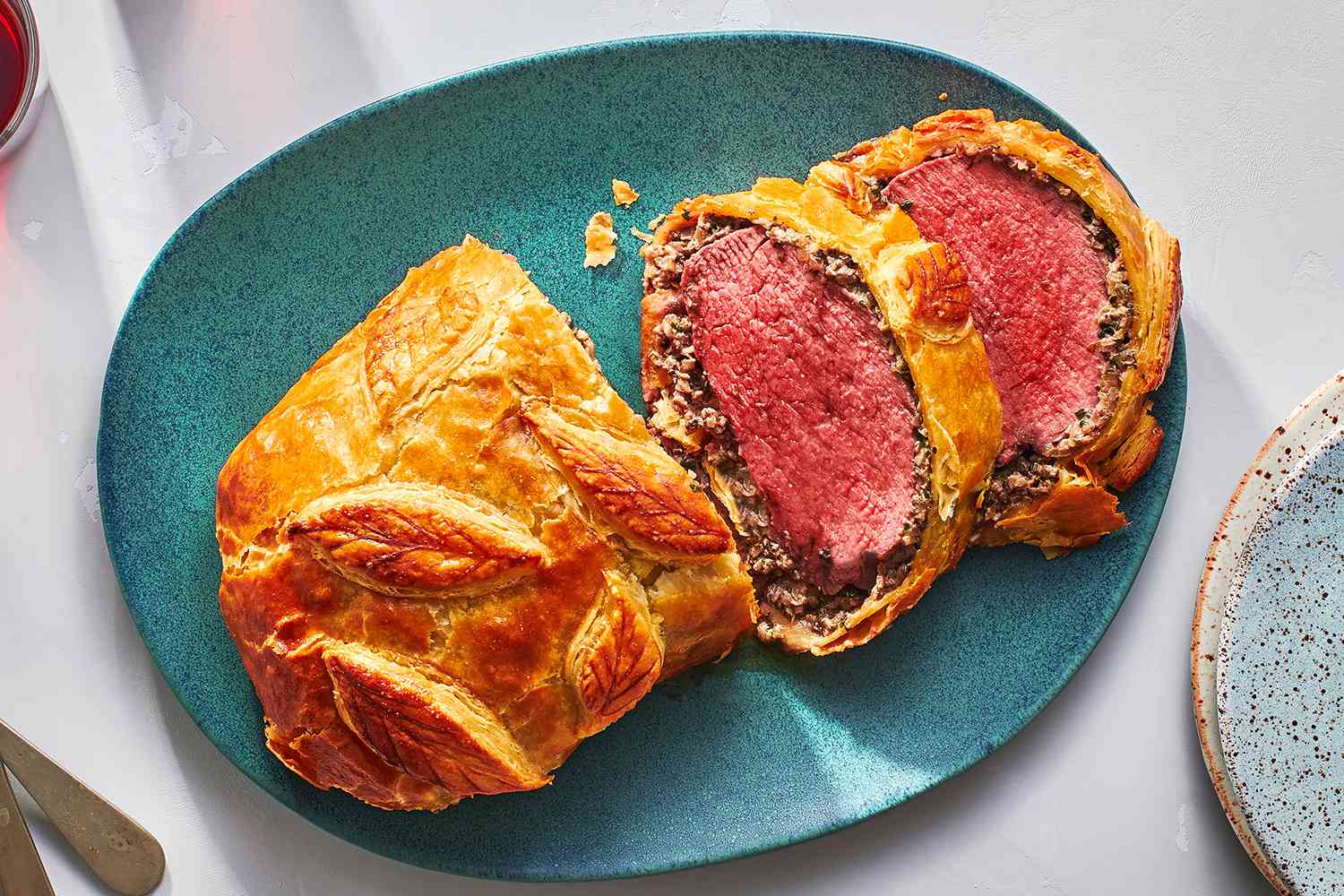The image captures a beautifully presented Beef Wellington placed on a speckled teal and blue oval platter. The photograph, taken from a top-down perspective, showcases the dish in full landscape orientation. The Beef Wellington sits prominently in the center of the platter, revealing both its artistry and culinary precision. On the left side of the plate, the Wellington remains whole, displaying detailed, buttery, leaf-shaped carvings on its thin, flaky crust. The right side has been sliced to reveal a perfectly cooked medium-rare roast beef encased within the pastry. The table beneath the platter is white, providing a clean, contrasting backdrop that highlights the dish's colors and textures.